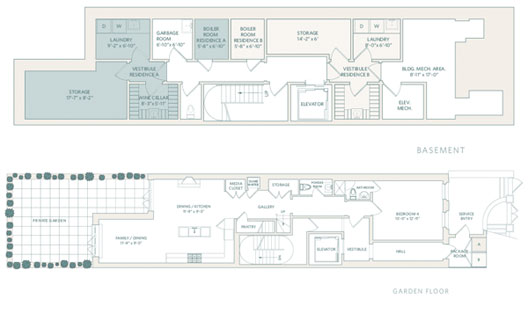Detailed Caption:

Here is a detailed blueprint of a multi-floor home, showcasing the layout and design of the basement and the garden floor. The blueprint is rendered in shades of tan and off-teal for enhanced clarity. The overall shape of the structure appears to be mostly rectangular.

The top section of the blueprint is labeled as "Basement." In this section, notable features include a designated laundry room, a large storage area, and a couple of staircases that provide access to the upper floors. 

The lower section is labeled "Garden Floor." This includes a beautifully designed garden patio, which integrates seamlessly with the indoor living space. The garden patio adds a touch of nature, enhancing the home's ambiance. The detailed layout offers a comprehensive look at the spatial organization and design aesthetics of each floor, despite the small and somewhat hard-to-read text.